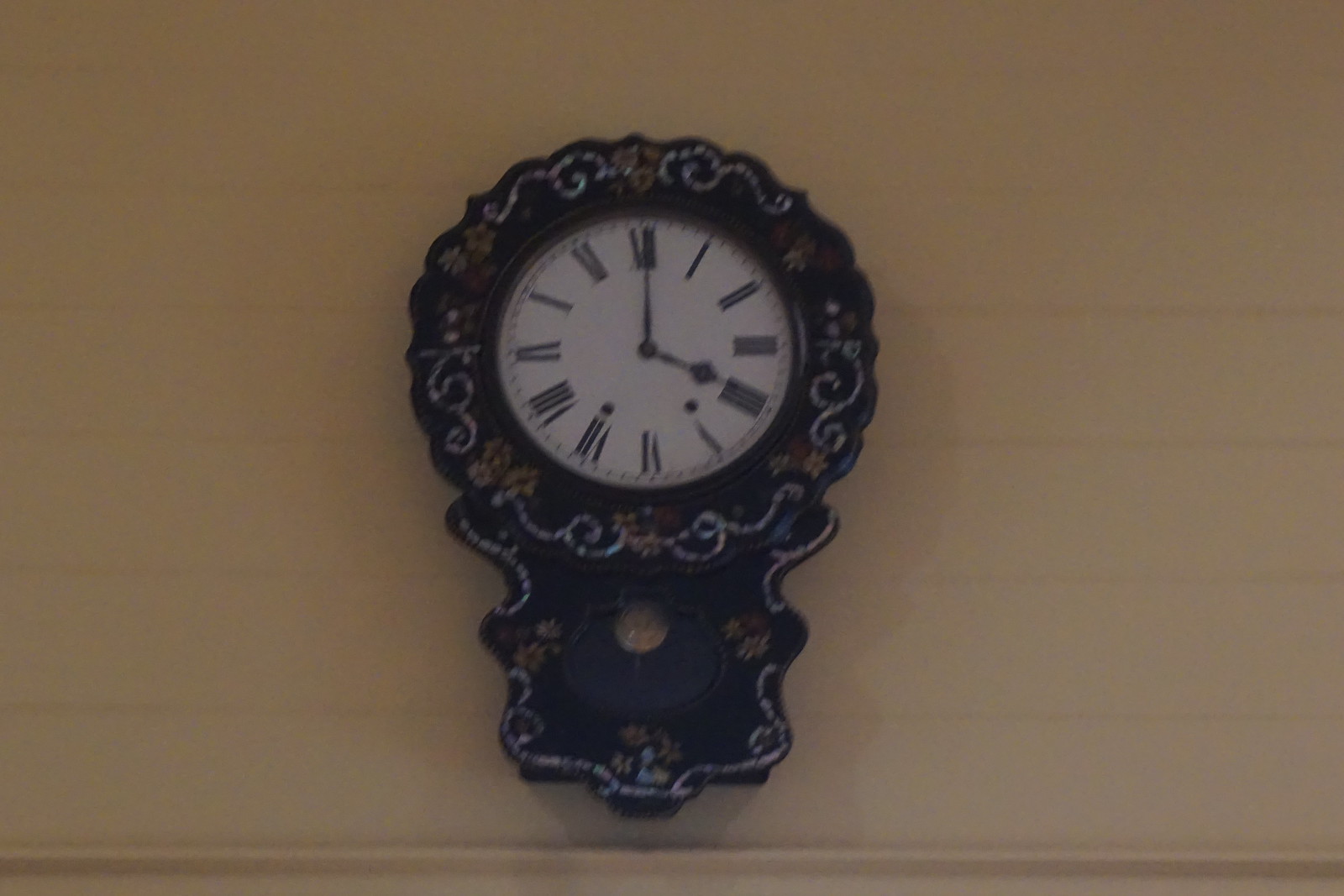This image depicts an antique-style clock mounted on a plain, horizontally-paneled beige wall. The clock is the sole adornment on the wall, emphasizing its vintage charm. The lower section of the clock is black, accented with an ornate white border. The circular face of the clock is encased in an intricately embellished, possibly floral, white frame. Below the clock face, a pendulum, reminiscent of those on grandfather clocks, can be seen oscillating. The clock face is white, adorned with black Roman numerals and black hands, indicating that the time is approximately three o'clock.